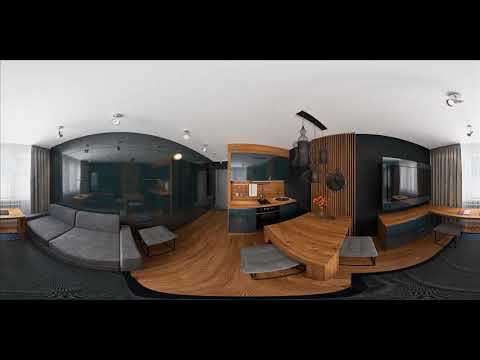The image is a wide panoramic view of a lavish, premium-designed room, cropped by thick black rectangles at the top and bottom. The white ceiling features multiple white lamps spread throughout. The left part of this expansive space showcases a large, gray, curved couch with two large cushions, accompanied by a side table. Adjacent to the couch is a window draped with a gray curtain. Behind the couch, there's a section possibly covered with black-tinted glass, reflecting parts of the room or providing a view through to another area.

The middle of the image features a light brown wooden floor, transitioning into darker tan shades leading to an entryway into a room resembling a kitchen. This kitchen area reveals details such as a dishwasher, rust-colored tile countertop, and potentially an oven. Further towards the center, a curved wooden table with two gray benches and a vase serves as an additional seating arrangement.

On the right side, the image displays an entertainment area with a large flat screen TV set against a black wall. Below the TV is a cabinet, with its top being brown wooden and the bottom part black. This section also includes another stool and a glass window with the curtain partially open, allowing natural light to filter through.